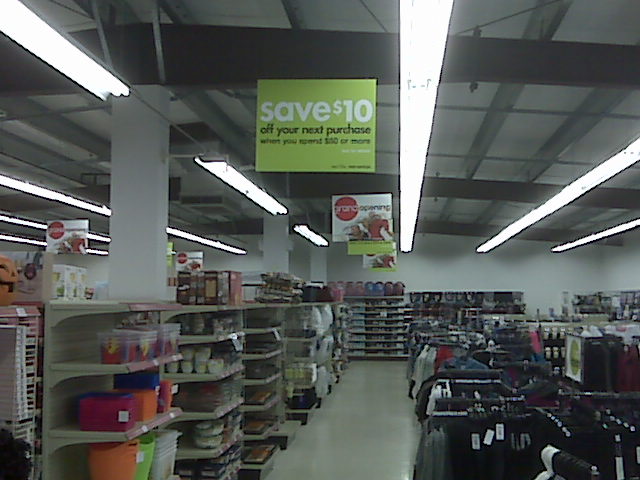The image depicts the interior of a retail store. On the right-hand side, there are racks filled with various clothing items, neatly arranged for customers to browse. On the left-hand side, multiple aisles are visible, each stocked with different types of home goods. One aisle appears to have storage containers, while the adjacent aisle seems to display dishes, cups, and bowls. Towards the back of the store, additional shelves with various products can be seen, although the details of these items are indistinguishable due to the distance. Hanging from the store’s ceiling is a prominent greenish sign that reads, "Save $10 off your next purchase when you spend $50 or more." Further in the background, another sign announces the "Grand Opening" of the store.